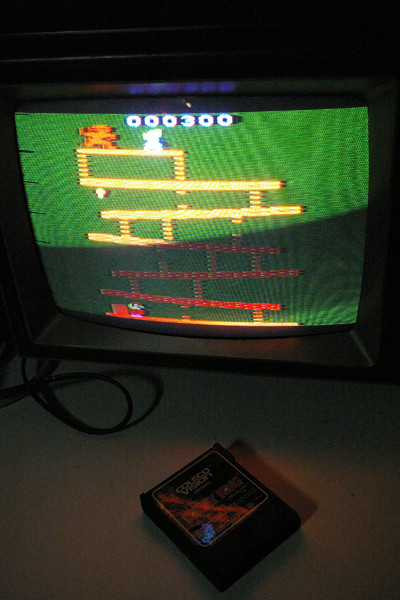This image captures a classic retro gaming moment, showcasing a photograph of a television screen displaying the iconic arcade game, Donkey Kong. The TV screen prominently features Mario at the bottom, beginning his climb up the series of red girders and ladders towards Donkey Kong and the captive princess positioned at the top of the screen. The score displayed reads "000300," indicating the points accumulated so far. The background of the game itself is a distinctive green, overlaid with the winding paths Mario must navigate. A shadow partially obscures the TV screen, adding to the nostalgic, slightly dim ambiance of the scene.

The TV has a bulky, black bezel, characteristic of older models, and visible at the bottom left corner are some attached cables, hinting at the connections required for this gaming setup. Resting on a white table beneath the TV is a black cartridge, which appears to be for a ColecoVision console, further emphasizing the vintage gaming theme. The overall atmosphere of the photograph is quite dark, enhancing the sense of being in a room filled with the intense focus and enjoyment of classic gaming.